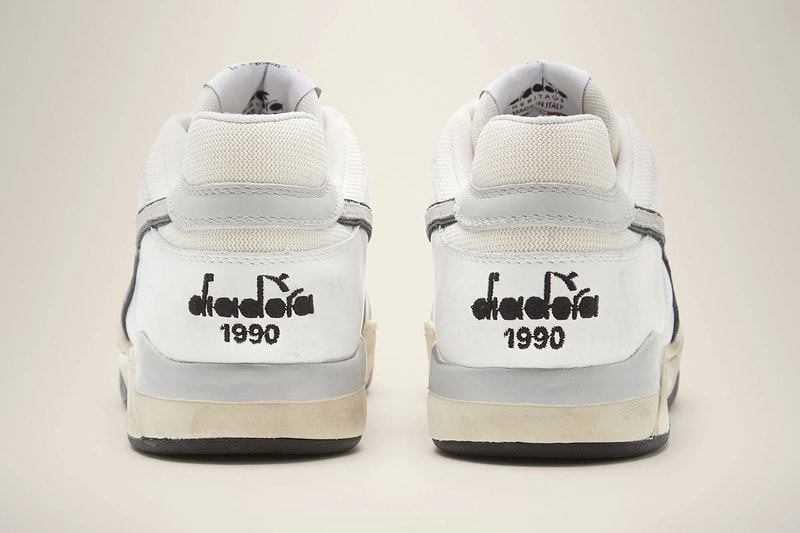This image showcases a close-up view of two white and gray sneakers, specifically from the back heel perspective, set against a white or off-white background. The shoes are positioned side by side, with their brand logo “Diadora” prominently displayed on each heel, along with the date “1990” underneath. These sneakers, adorned with various shades of white and gray, are constructed from a combination of different fabrics including mesh and possibly leather or faux leather. The midsoles of the shoes are white, contrasting with the black outsoles. Additionally, you can glimpse a part of the shoe tongues, which read “Diadora Heritage made in Italy,” indicating their Italian craftsmanship. The overall image is simple yet detailed, highlighting the fashion-forward and intricate design of the sneakers.